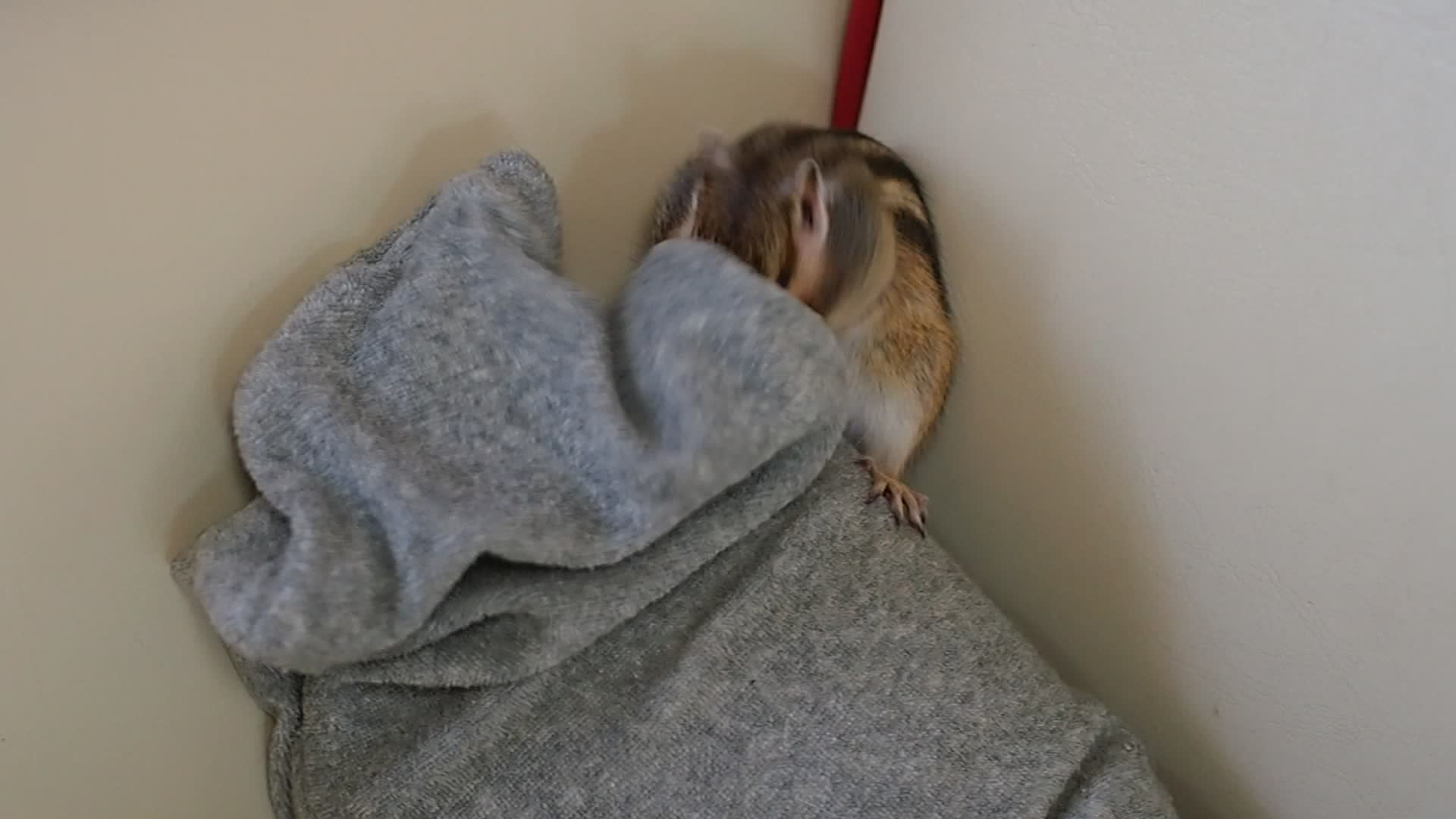In this landscape-oriented color photograph, a visibly healthy, chunky chipmunk with full cheeks is captured in the corner of a white-walled room. The chipmunk’s brown fur is accentuated with distinctive black and white stripes running down its back. Its small rounded ears peek out as it buries its face into a gray knit fabric, possibly part of a hoodie or sweatshirt, which is wadded up in the corner. The little creature's arched back and visible hind foot gripping the gray cloth suggest its quick movements, resulting in a blurred face. A red item, perhaps a leash or stick, is partially visible in the background, adding a pop of color to the scene’s clean, white surroundings where a vertical brown trim separates the two intersecting walls.